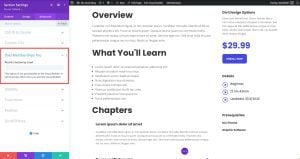In this visually engaging image set against a white background, multiple sections provide a detailed overview and valuable information. At the top, there's an overview section that introduces the topic, followed by "What You'll Learn" which includes a clearly formatted bullet list. The chapters of the content are outlined below this introductory area.

On the mid-right side of the image, there is a large purple rectangle alongside a black rectangle, each containing pertinent details about the subject matter. Additional information is highlighted within a prominent red rectangle.

At the bottom, four colorful squares draw attention with their distinctive hues. Each square—red, purple, blue, and green—features a unique white symbol or icon, though the specifics of these symbols are unclear. Near these squares, the price "2999" is written in blue text.

Complementing the design is a blue rectangle with white text, likely presenting a call to action or important message. Lastly, a purple circle is visible within the composition, further enhancing the visual appeal and organizational structure of the image.